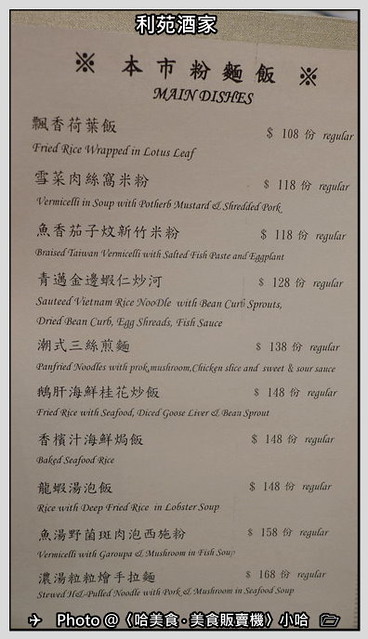Photograph of an Asian Restaurant Menu in Japanese or Chinese

This image captures a restaurant menu, prominently featuring characters in either Chinese or Japanese at the top, written in bold black font. Below the initial text, the words "Main Dishes" appear written in a stylish black cursive font. The top and bottom of the menu include watermarks consisting of white Asian symbols. At the bottom, there is an airplane-like icon followed by more white characters that likely provide additional context or branding.

The menu items listed include:
1. Fried Rice Wrapped in Lotus Leaf
2. Vermicelli and Soup with Pot Herb Mustard and Shredded Pork
3. Braised Vermicelli with Salted Fish Paste in Eggplant
4. Sautéed Vietnam Rice Noodle with Bean Sprouts
5. Dried Bean Crab Egg Salad with Fish Sauce
6. Noodles with Mushrooms, Chicken, and Sweet and Sour Sauce
7. Fried Rice with Seafood, Diced Goose Liver, and Bean Sprouts
8. Baked Seafood Rice
9. Rice with Deep Fried Rice and Lobster Soup
10. Mushroom Soup
11. Noodle Pork Mushroom and Seafood Dish